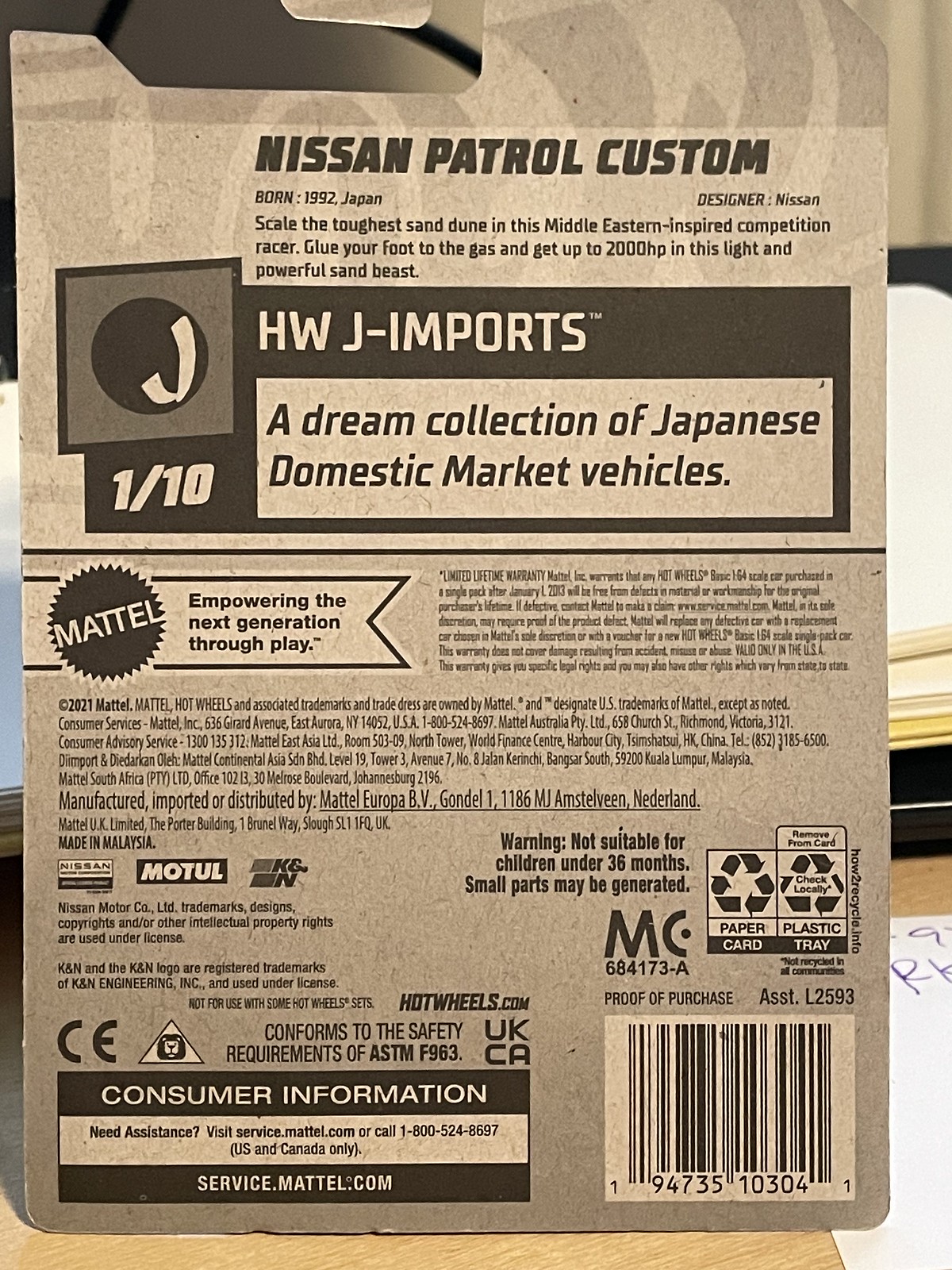This image depicts the back of a toy car package, resting on a light brown table or desk, accompanied by a white sheet of paper with illegible scribbles and possibly a book or file in the background. The rectangular packaging, which appears to be made from a recycled brown-gray cardboard, features an array of detailed product information and branding elements.

The top of the packaging prominently displays "Nissan Patrol Custom" in bold black letters. Directly below, it reads, "Born 1992, Japan. Designer: Nissan. Scale the toughest sand dune in this Middle Eastern-inspired competition racer. Glue your foot to the gas and get up to 2,000 HP in this light, powerful sand beast."

Under this description, the text continues in a black box with white letters, stating "HWJ Imports." Beneath this is another white box containing the phrase "A Dream Collection of Japanese Domestic Market Vehicles." To the left is the HWJ Imports logo, consisting of a white "J" inside a black circle, which is set within a gray square with black borders.

Adjacent to the logo, the text "1-10" indicates that this is item one of ten in a collection. Additional logos include a spiked emblem with the word "Metal" enclosed in a ribbon-shaped box, accompanied by the slogan, "Empowering the Next Generation Through Play."

The bottom section of the packaging is dense with fine print, including legal text, brand logos, and various consumer information. The Mattel logo appears with detailed contact information for different global locations including the USA, Australia, Hong Kong, Malaysia, South Africa, the Netherlands, and the UK. There are also logos for Nissan, Motul, K&N, and additional trademarks for Nissan Motor Co., K&N Engineering Inc., and Hot Wheels.

The barcode, located at the bottom right corner, includes the numbers "9473510304" and the words "Proof of Purchase ASST.L2593." Safety warnings state that the product is not suitable for children under 36 months due to small parts. Further details include recycling information, conformity symbols such as UKCA and CE, and the statement, "Confirms to safety requirements of ASTM F1063."

In summary, this detailed toy car package back cover emphasizes extensive branding and legal information, designed to assure quality and safety compliance.